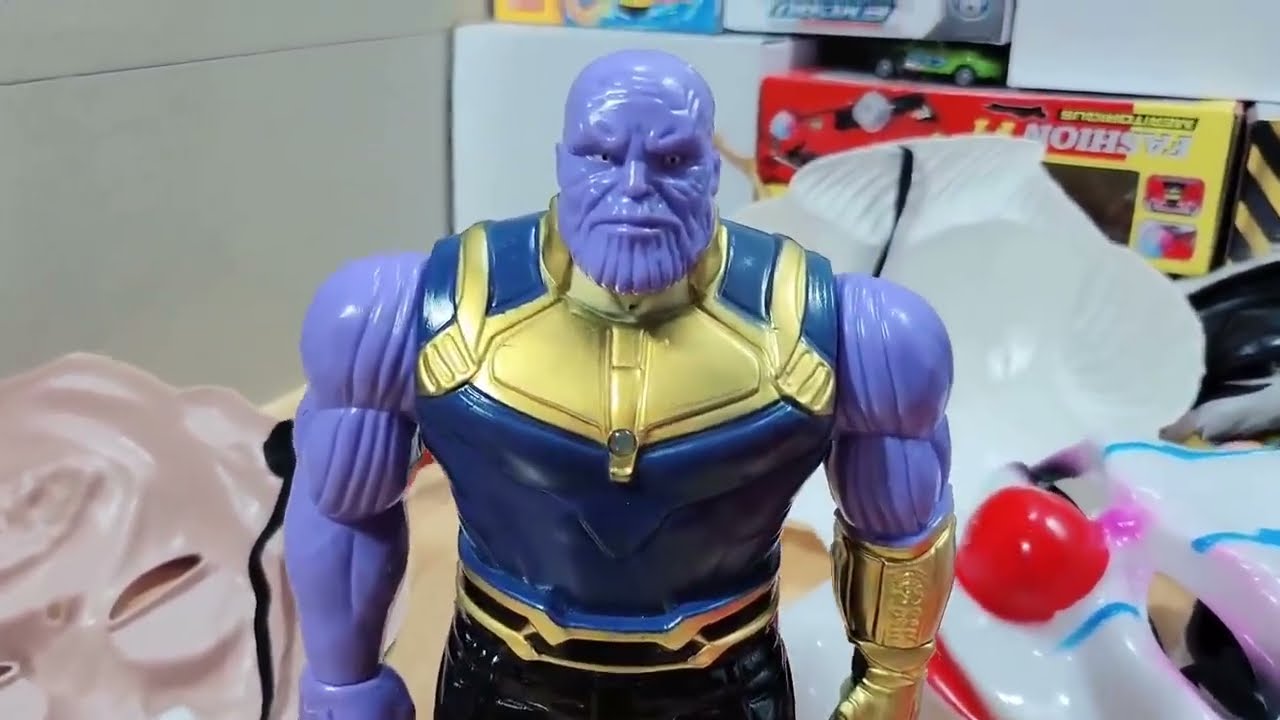The image features a close-up of a Thanos action figure, primarily shown from the waist up. This plastic figure is bald and has a light purple complexion with muscular exposed arms. He is outfitted in a blue sleeveless shirt with a distinctive gold collar, complemented by dark-colored pants. His left hand is adorned with the iconic gold Infinity Gauntlet that stretches up to his elbow. In the background, there is a collection of various toys, including a box that appears to contain an upside-down remote control car and some generic packaging. Notably, several upturned plastic Halloween masks are visible, showing their insides, while to the right of Thanos, a white clown mask with a red nose and blue stripes is facing forward. The scene is set against white walls, resembling office dividers, emphasizing the cluttered but intriguing backdrop.